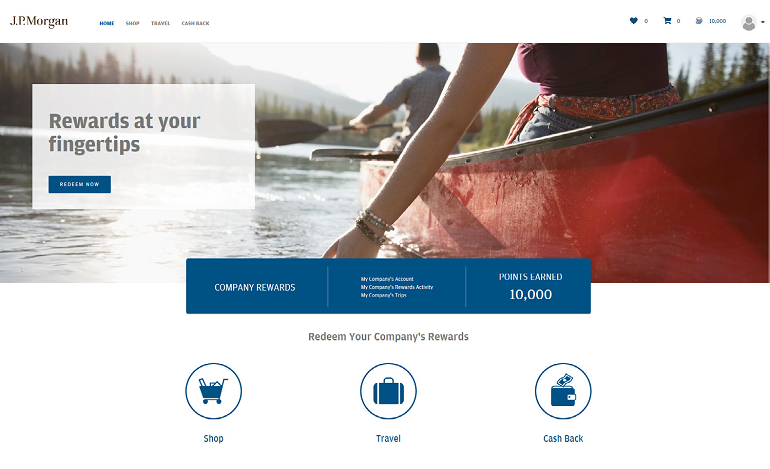The image displays a webpage from JP Morgan, identifiable by the black "JP Morgan" text prominently positioned at the top left corner. The site is neatly organized into categories, colored and labeled as follows: "Home" in blue, "Shop," "Travel," and "Cashback". The main banner headline reads "Rewards at your fingertips" with a "Redeem Now" call-to-action button positioned below.

A picturesque image of a man and a woman in a boat, with the man rowing, adds a personal touch to the page. In the top right corner of the page, various icons with accompanying statuses are displayed: a like icon showing zero likes, a cart icon indicating an empty cart, a credits display showing a balance of 10,000 credits, and a user icon representing the account section.

Further, specific details such as "Company Rewards," "My customer's account," "My company's rewards," and "My company's trips" are listed alongside the points balance of 10,000. Additional options like "Redeem your company rewards," "Shop," "Travel," and "Cashback" are also integrated to guide the user through possible redemption options.